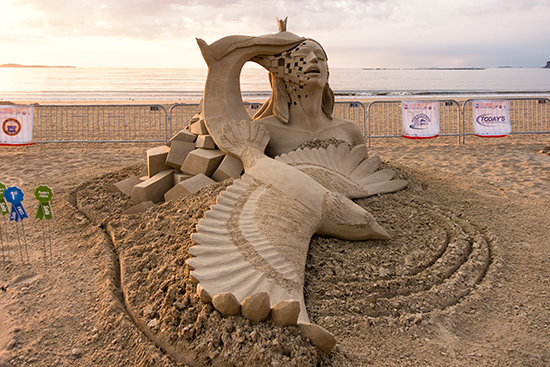This photograph captures an intricate sand sculpture on a sandy beach. At the center of the scene is an eagle crafted from sand, lying flat with its wings outspread, constructed from darker sand for the body and lighter sand for the wingtips. The eagle is depicted with its head down and tail pointed up, showcasing detailed feather ridges. Emerging from behind the eagle is a mermaid rising from blocks of sand. She has long, flowing hair and a mermaid tail that bends over her head. Small squares are cut out of her face, and her open mouth points skyward. Surrounding the sculpture is a guardrail, and in the background stands a wire fence adorned with white signs, beyond which lies the beach's expanse, the ocean, and clouds in the sky. To the far left, ribbons, including a first-place ribbon, are visible, adding to the scene's detail and overall composition.